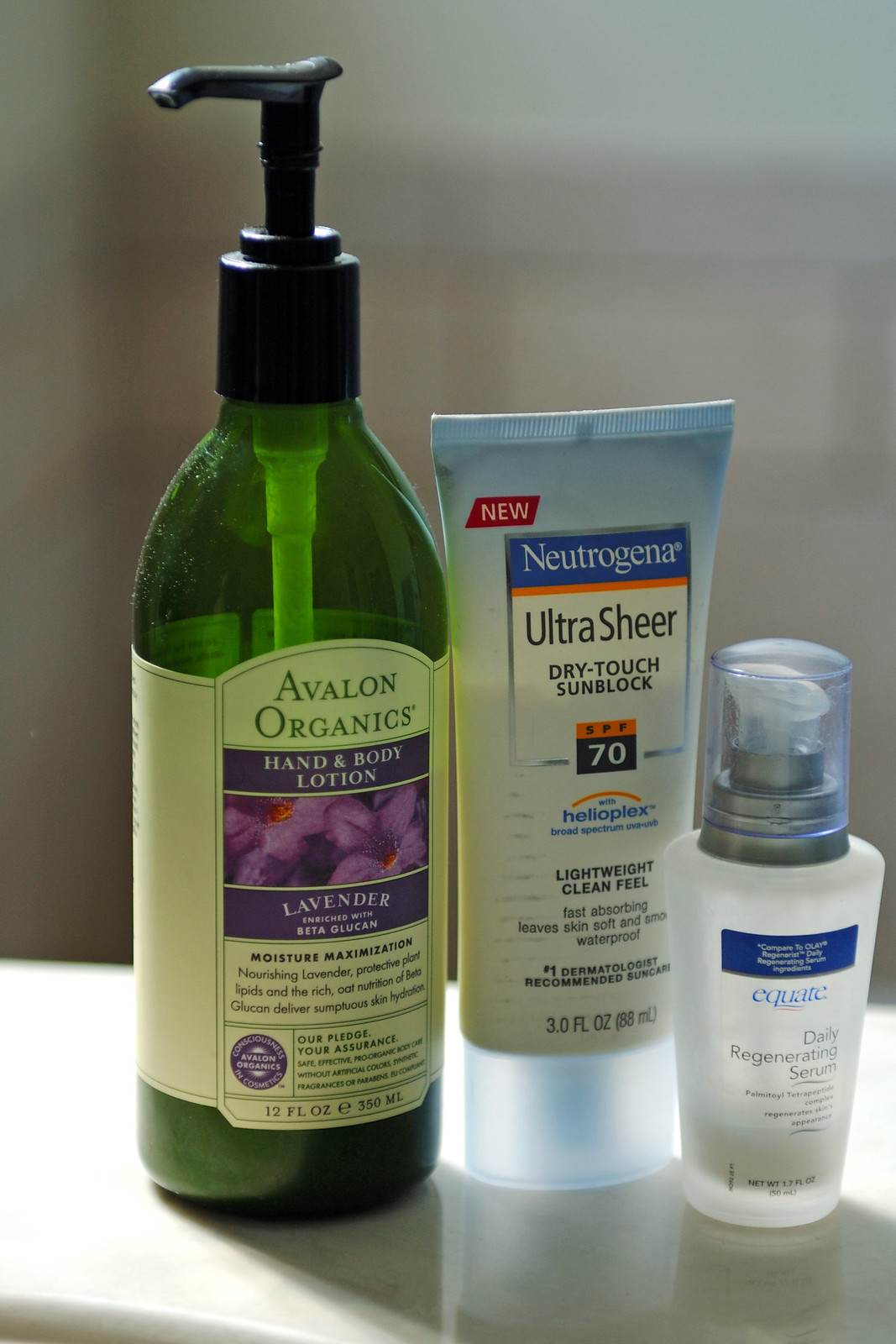On the shelf, a collection of cosmetics is neatly arranged. To the far left sits a bottle of Avalon Organics hand and body lotion, encased in a green-colored glass with a black pump handle at the top. The bottle features a lavender scent and is specifically designed for moisture maximization, with text highlighting that nourishing lavender provides rich moisture. A purple seal adorns the bottle, and at the bottom, it's denoted that it contains 12 fluid ounces.

Adjacent to the lotion is a tube of Neutrogena Ultra Sheer Dry Sunblock boasting an impressive SPF of 70. Labeled as "new" at the top, the sunblock promises a lightweight and clean feel, with additional text noting it as the number one dermatologist recommendation. The packaging is predominantly white, accentuated with a clear, translucent cap, and contains 3 fluid ounces of product.

The third item is a frosted bottle of Equate Daily Regenerist Serum. This product features a pump handle topped with a dark gray cap, and it is further protected by a clear outer cap. The slender, translucent bottle reveals a white liquid inside, reinforcing its purpose as a rejuvenating serum.